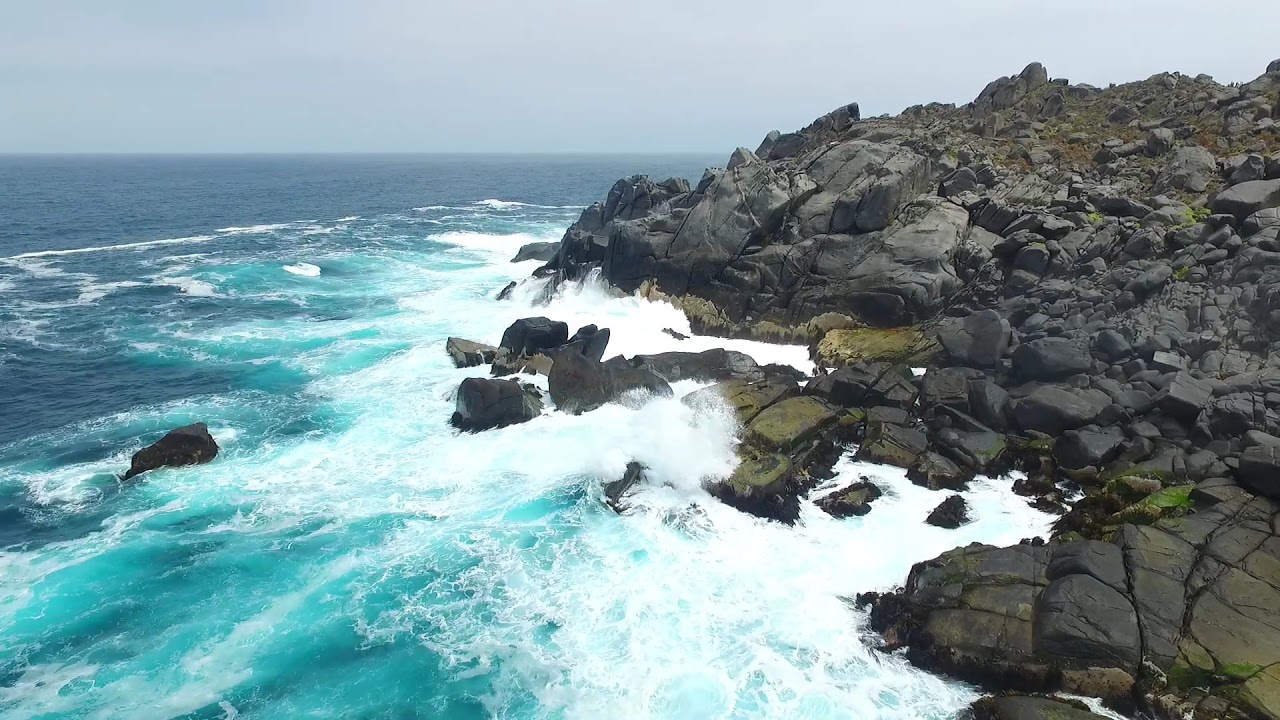The photograph captures a rugged shoreline where the powerful ocean meets the rocky coast. On the left side, the expansive ocean is a dark blue that gradually lightens as it approaches the rocks on the right side, eventually turning white as the waves crash against the shore. The right side of the image features numerous dark gray rocks covered in green moss, creating a textured contrast. Sparse vegetation can be seen on these rocks, which form a hill as they recede into the background. The shore itself is devoid of sand, composed entirely of rocks and large boulders. The sky above is a dark, hazy gray, adding to the dramatic and powerful atmosphere of the scene. The image is devoid of any human presence, emphasizing the raw, natural beauty and tranquility of the coastline.